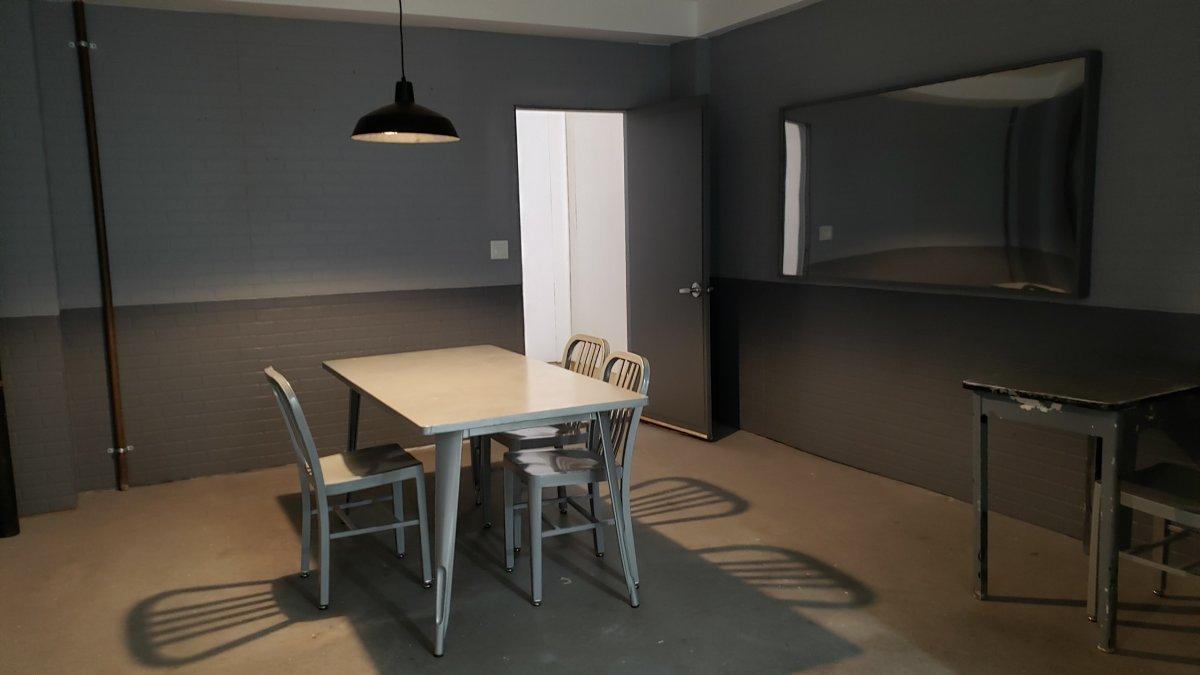This image depicts a stark and intimidating interrogation room. At the center, a light gray table with four slightly outward-facing legs stands under a harsh overhead light, emitting a yellow-tinted glow from a black-cased fixture suspended by a thin cord. Around the table, there are three silver metal chairs, one on the left and two on the right, each casting elongated shadows with four-bar details and oval shapes. The room's walls are made of brick, painted with light gray on top and dark gray below, while the floor has a tan or gray concrete finish. In the background, an open black security door with a silver handle reveals a lighter colored hallway with white walls. To the far right, a large rectangular one-way mirror embedded in the wall reflects the room's details, emphasizing its function as an interrogation space. Near the bottom right corner, there's an old, dark brown table with chipped paint and a lone chair, enhancing the room's overall atmosphere of disrepair and unease.